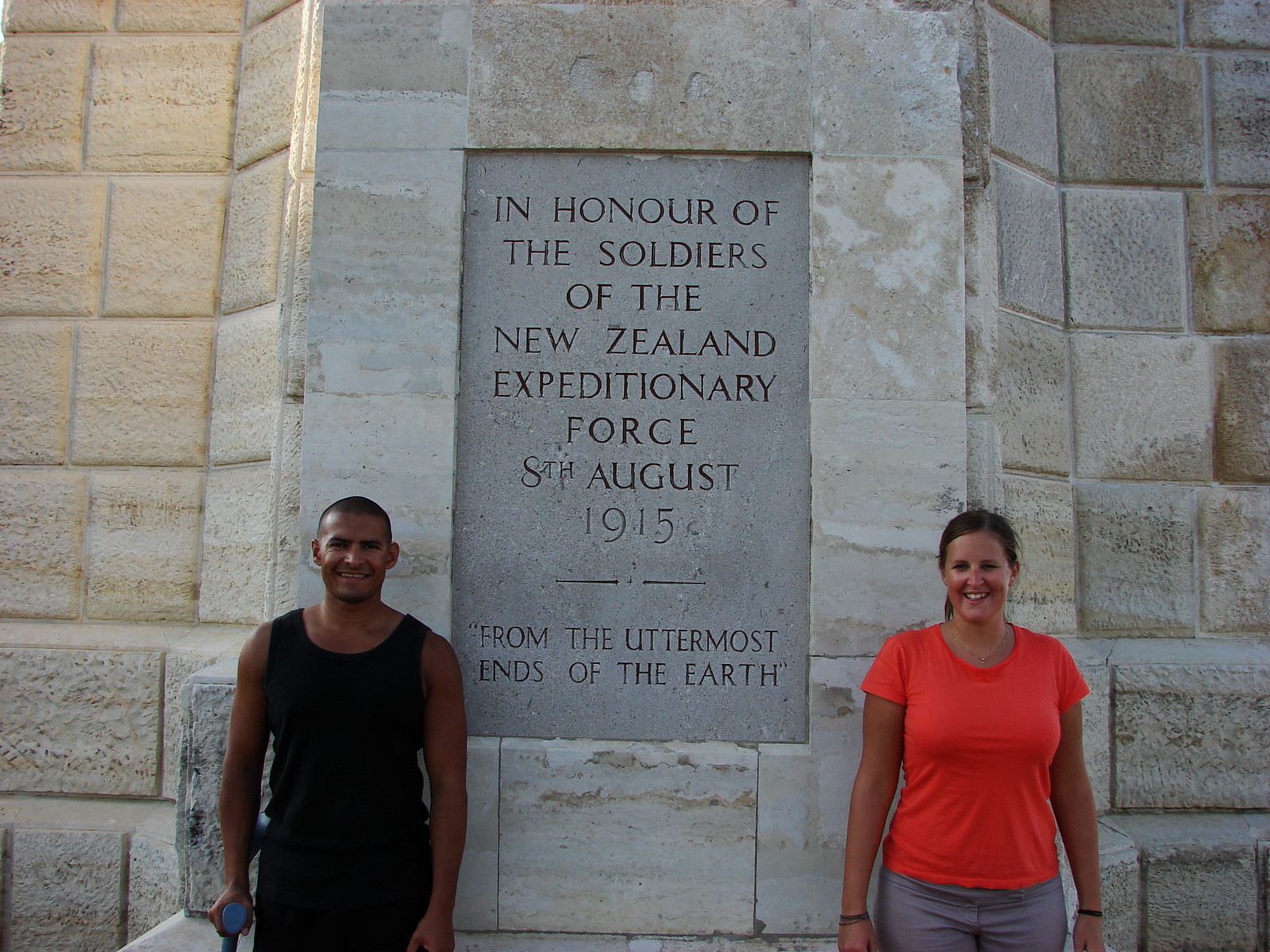The photograph captures two smiling individuals posing on either side of a large, white sandstone monument. The central feature of the monument is a recessed grey stone placard with carefully carved letters that read: "In honor of the soldiers of New Zealand Expeditionary Force, 8th August 1915. From the uttermost ends of the earth." The man on the left is visible from the waist up, sporting black pants and a sleeveless black tank top. He has very short, black hair and is holding a blue bottle in his right hand. The woman on the right is visible from her upper thighs and has brown hair pulled back into a ponytail. She is dressed in grey pants and a short-sleeved orange top, accented with bracelets on both wrists. She is looking slightly downward to her right, enhancing her cheerful expression. Both individuals are dark-skinned and stand against the monument's expansive, distinctively white and grey marbled surface.